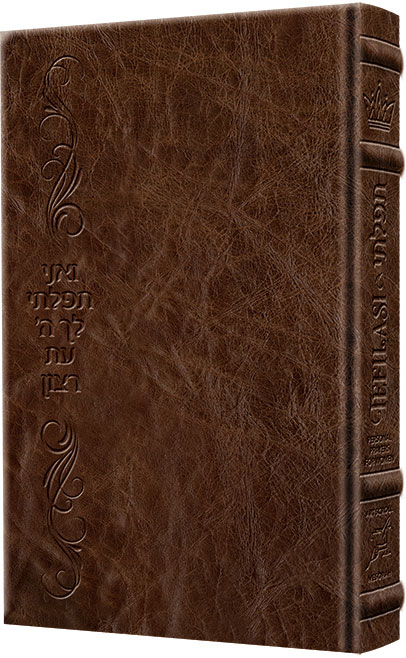This photograph features a tall, brown leather hardcover book set against a stark white background. The image captures what is believed to be the back cover of the book, which is adorned with ornate, etched designs. The binding, visible on the right side, also showcases intricate engravings, including a decorative motif that resembles a crown. Despite these unique details, the text on the book is unreadable and appears to be in either Hebrew or Arabic, although it is challenging to determine definitively. No additional identifying information, such as the book’s title or publication year, is discernible. This image closely resembles a stock photo, presenting the book in a simple and isolated context.